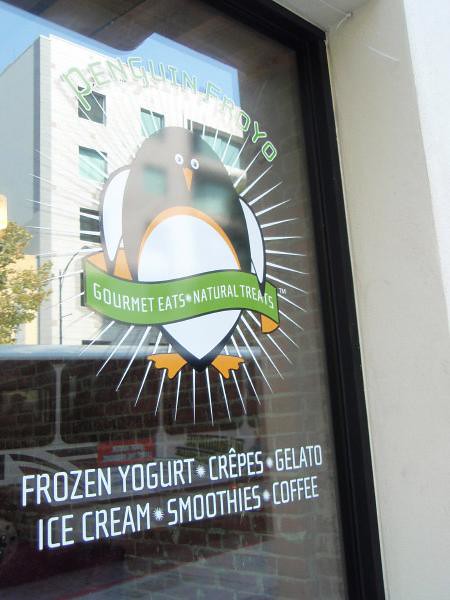This daytime photograph captures the inviting storefront of "Penguin Froyo." Prominently displayed on the window is the store's logo, featuring a teardrop-shaped cartoon penguin adorned with a yellow U-shaped pattern on its chest. The penguin is emblazoned with a sash bearing the trademarked phrase, "Gourmet Treats, Natural Treats." Above this lively character, the store's name, "Penguin Froyo," is written in green text. Below the penguin, a list of delightful offerings appears in white text: frozen yogurt, crepes, gelato, ice cream, smoothies, and coffee. The window's reflection reveals a four-story geometric office building, a clear blue sky, a tree, and a bus parked outside, suggesting a bustling urban environment. The storefront's brick interior wall and the vibrant colors of light green, black, dark green, dark brown or red, and blue, further enhance the lively ambiance of this gourmet treat shop.